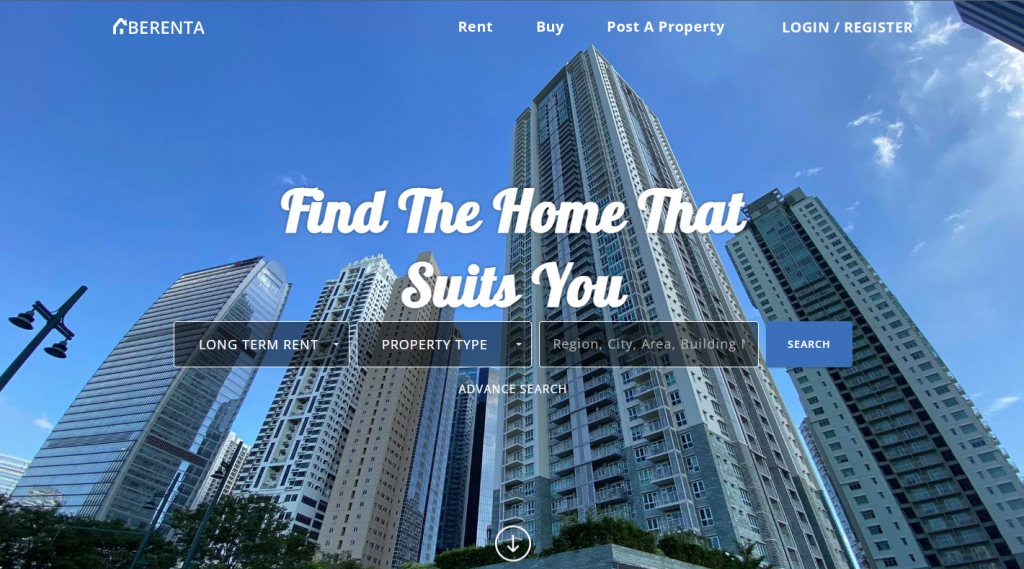Photographed from the ground looking up, this image showcases towering skyscrapers that appear to be residential apartments, evidenced by the numerous balconies adorning each floor. The vastness of the buildings is emphasized by their height, reaching towards a picturesque sky painted in vibrant shades of blue, dotted with a handful of fluffy white clouds. Prominently displayed over the image is the website "Berenta", advertising options to rent properties. The overlay includes commands such as "Rent by", "Post the property", and "Log in / Register". A bold headline across the skyscrapers reads, "Find the home that suits you". The interface also features multiple interactive elements: black boxes with options for "Long-term rent", "Property type", "Region, city, area, building", and a blue search box. Additionally, there is an option for an "Advanced search" beneath these selections, accompanied by a downward-pointing arrow enclosed in a circle. This meticulously captured scene not only promotes the concept of urban living but also highlights the seamless integration of modern technology with everyday life.